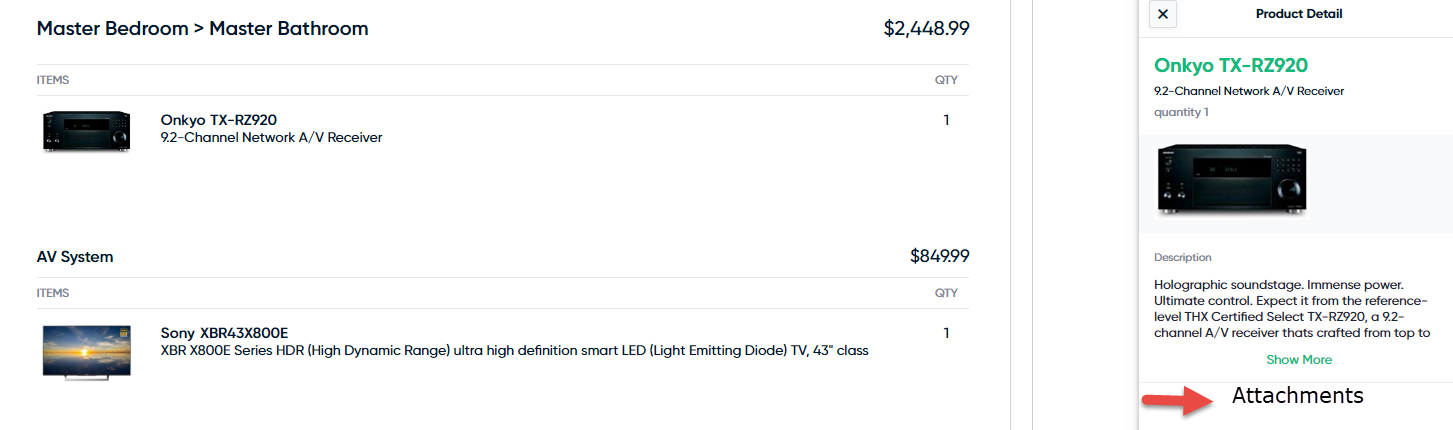Screenshot showcasing a detailed shopping list for a Master Bedroom setup. The image features a predominantly white background with several highlighted elements. The phrase "Master Bedroom" is prominently displayed with an arrow pointing towards another "Master Bedroom" label. The total cost is listed as $2,448.99. Additionally, there is a section labeled "AV," indicating an audio-visual system priced at $849. Also included is a high-end Sony TV with a screen size of 43 inches. There appears to be a channel network receiver, which has a descriptive arrow pointing to attachment details, enclosed in a paragraph. This component is black and marked with green text indicating product details. There is also an option to click "show more" for additional information.